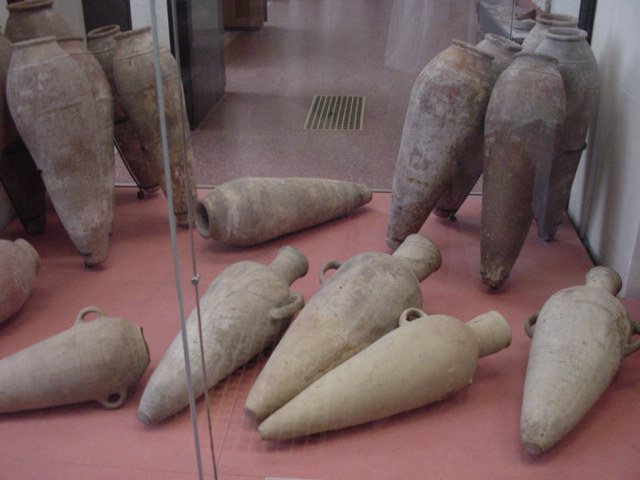This color photograph captures an exhibit of ancient-looking clay vessels in a museum display case. The vessels, potentially made from terracotta or earthenware, have a pointy, carrot-like shape tapering to a narrow tip, with small handles or ear-like grips near their tops. These handles suggest they might have been used for carrying liquids like water or wine. The vessels are arranged haphazardly within the glass case; some lie diagonally on their sides, while others stand upright, leaning against each other. The ones lying down are a light tan color, contrasting with the standing ones that are darker and appear dustier, bearing shades of brown, purple, and gray. The floor inside the case is a muted reddish-pink, tile-like surface, possibly ceramic. Reflections on the glass case indicate that the exhibit is part of a larger museum space with similarly tiled flooring and white and greyish walls. In the background, a grey grid drain is visible amidst the red flooring, adding to the impression of an organized but aged historical display.